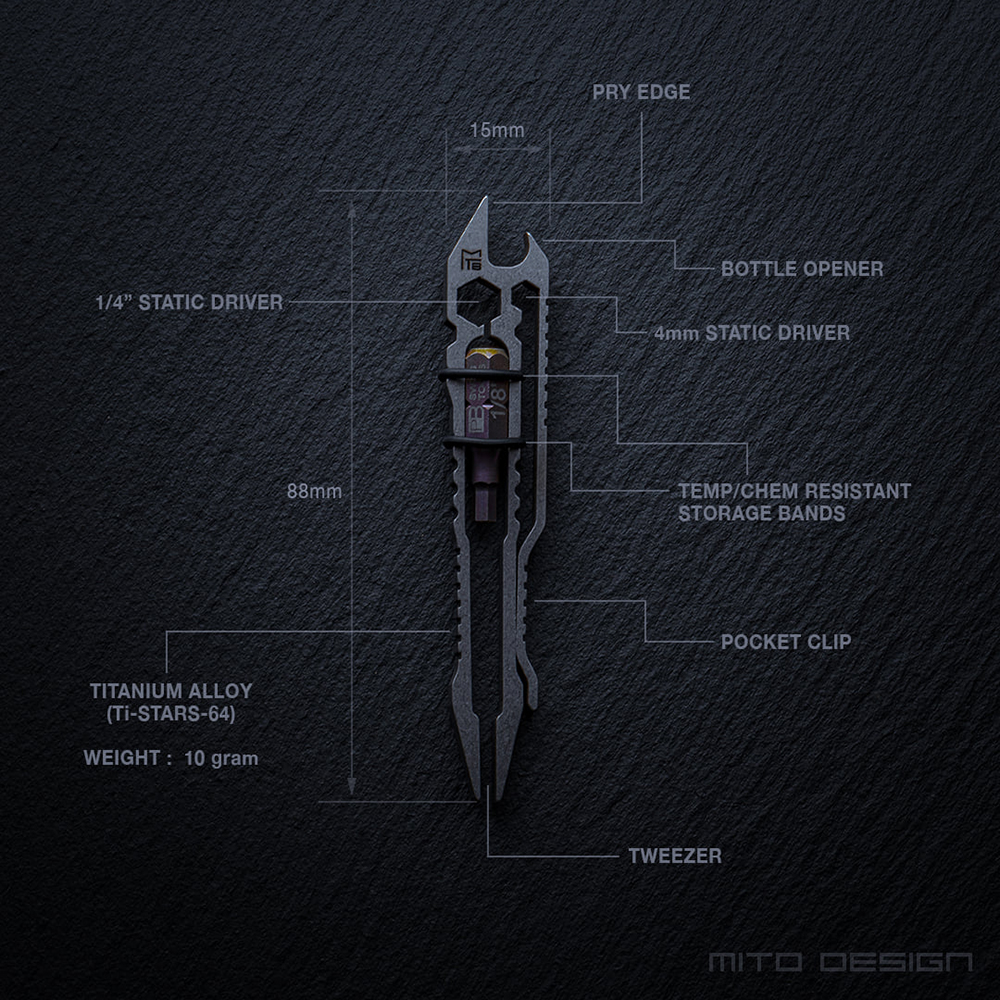The image depicts a multi-tool against a dark grey stone-like background with a diagonal grain, tapering horizontally shorter than vertically. The multi-tool is crafted from a dark grey metal and features various components, meticulously labeled with lines connecting to respective parts. Prominent text includes: "15 millimeter" width, "88 millimeter" height, "titanium alloy TI Star 64," and "weight: 10 grams." The tool includes a "pry edge," "bottle opener," "4 millimeter static driver," "TempKem resistant storage bands," "pocket clip," "tweezer," and a "quarter inch static driver." At the bottom right corner, "MITO DESIGN" is embossed in a machine-like font. This comprehensive labeling and detailed engineering suggest it's a sophisticated, compact multi-tool suitable for various functions.